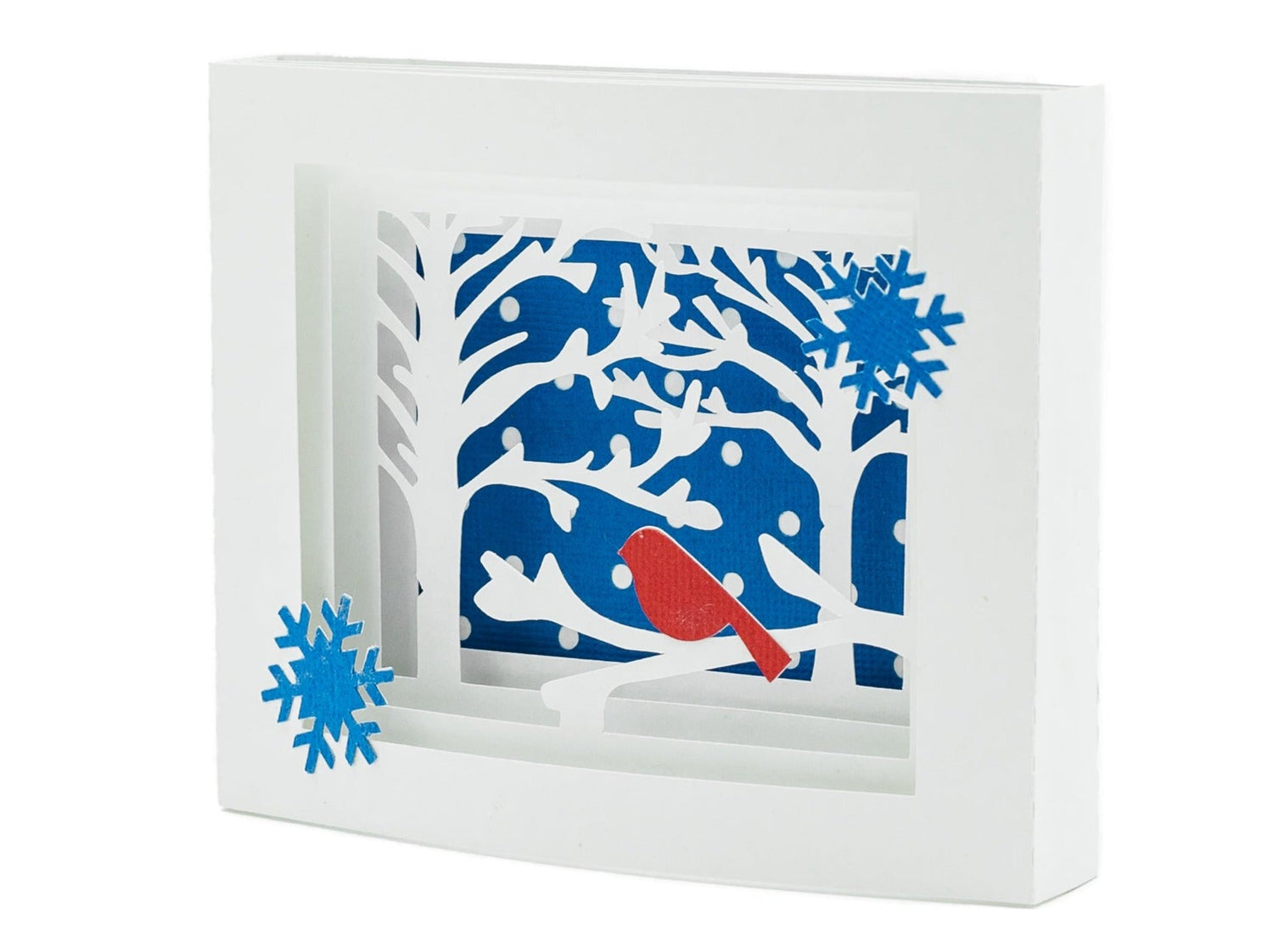The image is of a white object, likely a binder or box, standing upright against a solid white background. The front features a beautifully crafted winter scene, resembling an art project or greeting card with intricate cut-out layers. Dominating the center is a square blue background adorned with white circles representing falling snow. White tree branches extend across the blue, with a red robin perched delicately on one of them. There's a prominent blue snowflake in the top right corner and another in the bottom left. The scene is framed by light grey borders, enhancing the layered, three-dimensional effect, making the wintery tableau appear rich and detailed.